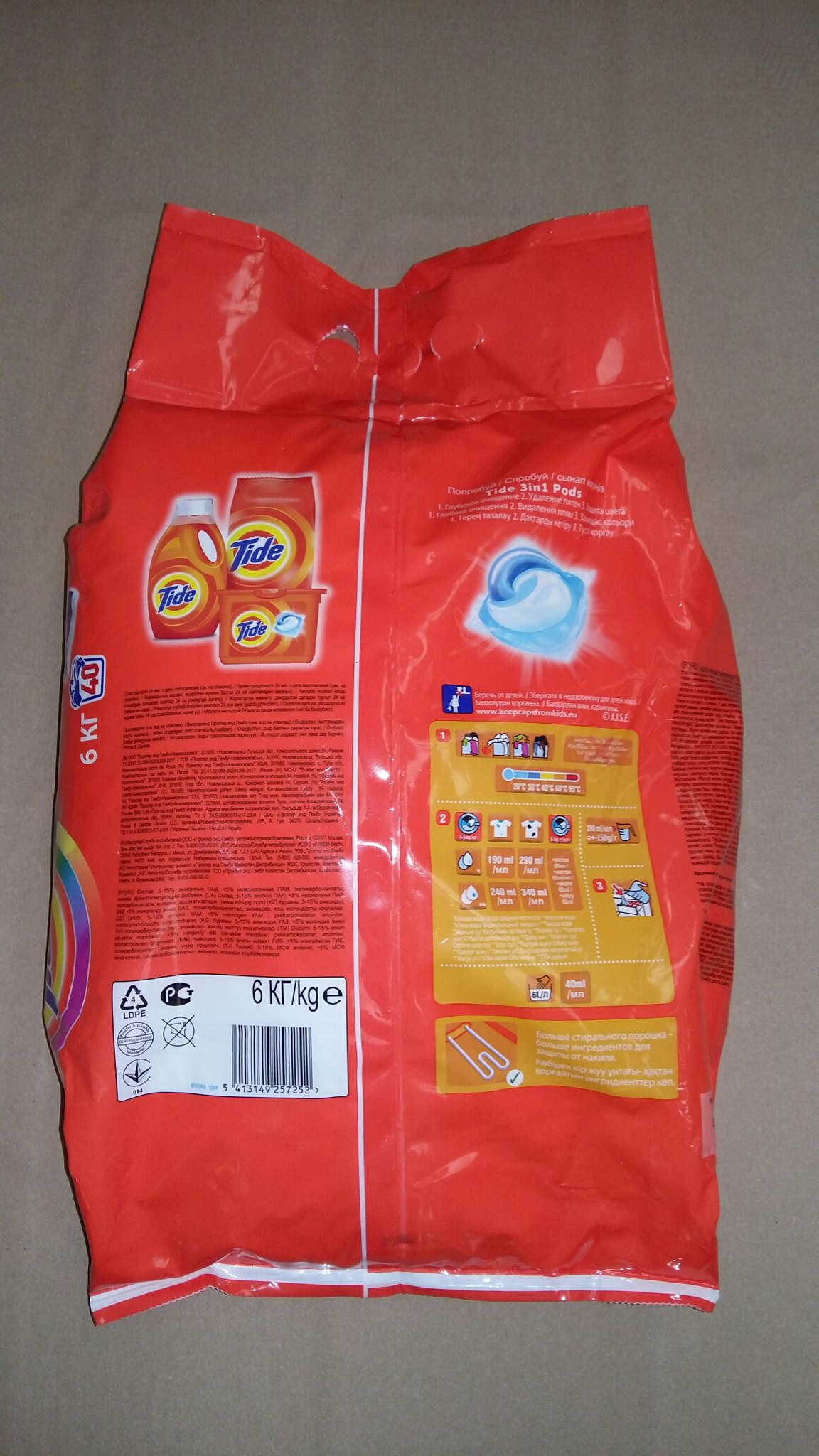This photograph captures an unopened red bag of Tide 3-in-1 Pods, prominently displaying its back side. The bag rests on a surface that appears to be either a white or light brown sheet—difficult to discern due to the lighting. The bag’s upper right corner features an image of a Tide Pod, depicting its distinct swirly design in cyan blue, white, and dark blue. Adjacent to this, the upper left side showcases different Tide products including the liquid, powder, and this particular bag of pods. A striking orange rectangle highlights multi-step washing instructions alongside an orange legend. Below these, a block of unreadable black text occupies the left-hand area of the bag, accompanied by a white box containing the UPC code. The bottom right corner also displays a symbol of a laundry basket with clothes and the number 40 encircled by blue lines. The encompassing gray background suggests a countertop beneath the bag.